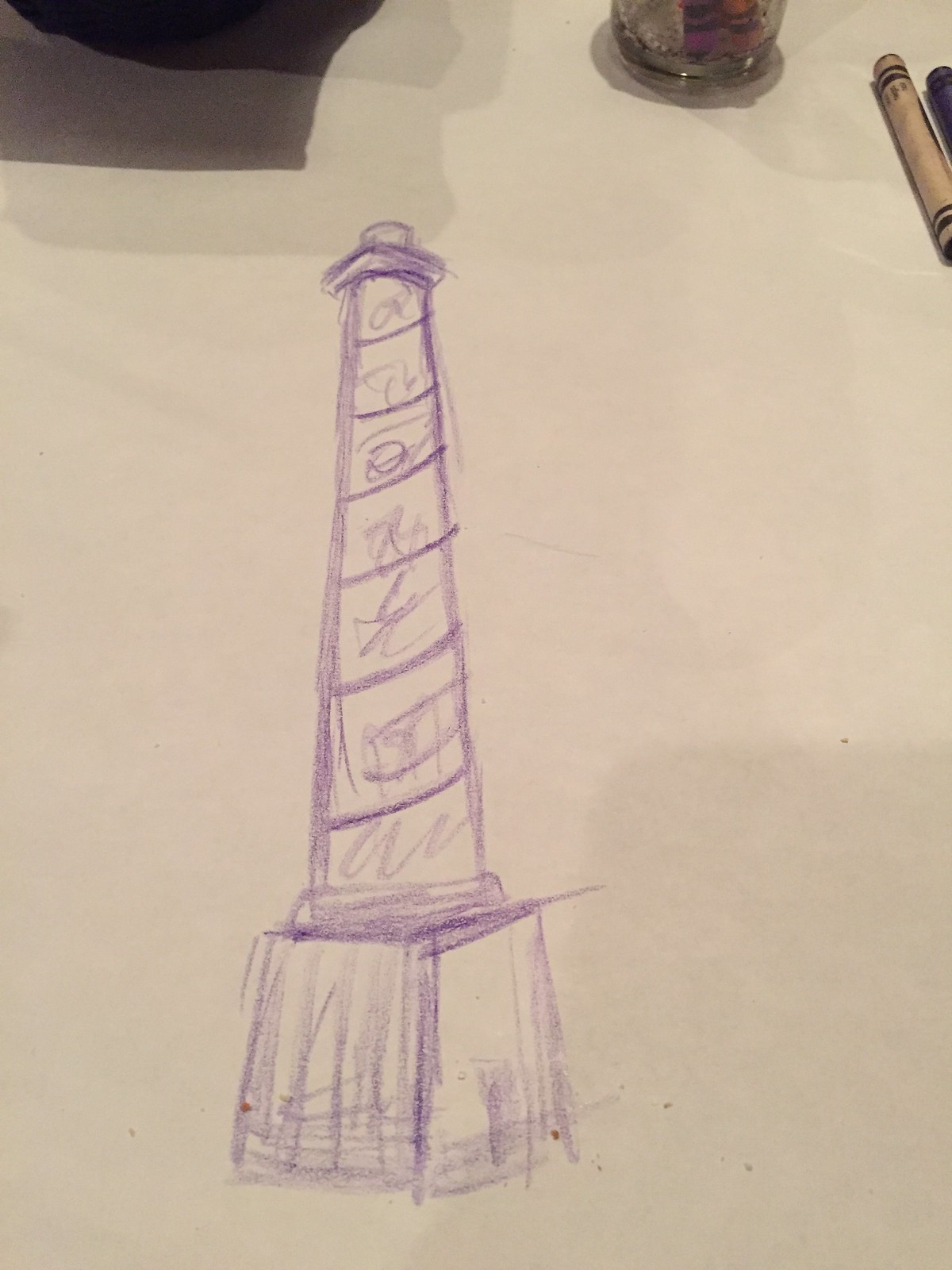A child's crayon drawing on a white sheet of paper. The drawing is somewhat sloppy, indicative of a young artist's hand. In one corner, a glass cup holds a purple and a reddish crayon, while two more crayons are partially visible beside it. The main subject is a lighthouse-like structure with a thick base, adorned with stray crayon marks and scribbles. The lighthouse features a striped pattern ascending its height, topped with a square section and crowned with a circular dome. Gray shadowing adds depth to the image. At the very top, a dark-colored object is present, but its details are indistinguishable.